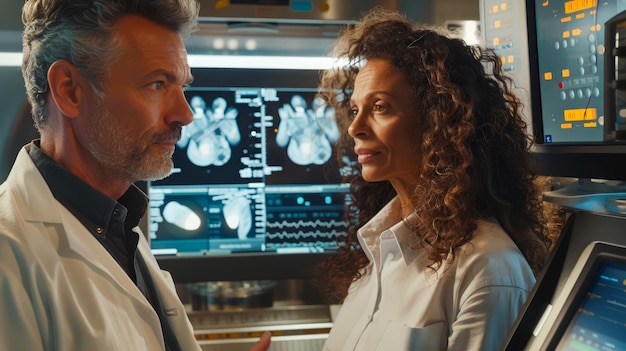In this detailed photograph, we see a scene reminiscent of a medical drama, featuring two individuals who might be doctors or scientists. The male figure on the left, sporting short hair, a gray-and-white beard, and a black shirt beneath his white lab coat, gazes intently at a screen on the right side of the image. The female figure on the right, who has curly hair and wears a white collared button-up shirt with a front pocket, looks slightly confused and is staring towards the male doctor. Surrounding them are various monitors and complex medical equipment, adding to the sophisticated lab setting. One prominent screen in the background exhibits ultrasound-type images in four quadrants, contributing to the clinical atmosphere of the scene. Both individuals appear to be engaged in a serious moment, enhancing the gravity of the situation depicted.